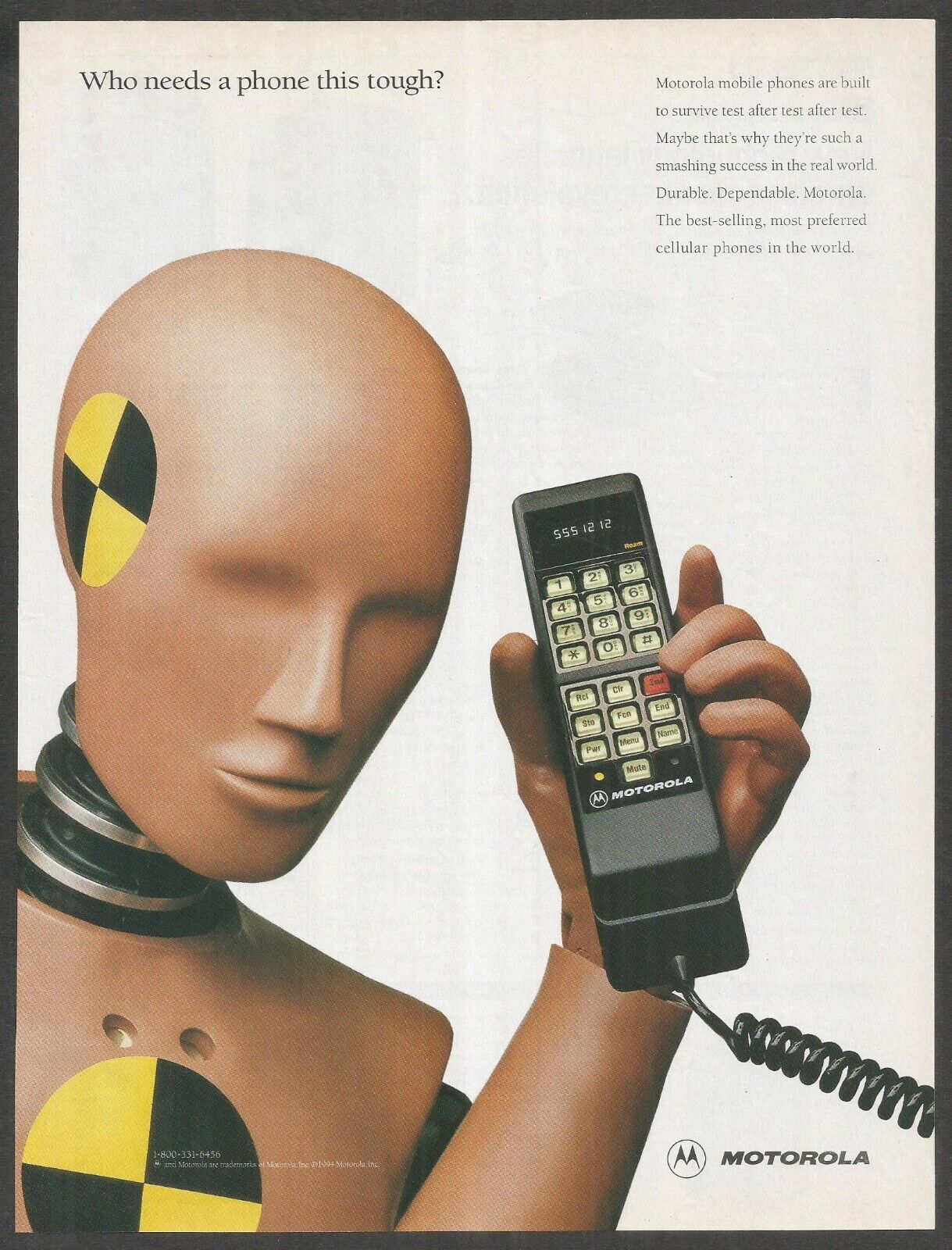This image is an advertisement, likely from a magazine in the late '80s or early '90s, showcasing a Motorola mobile phone. The ad features a slightly browned, old paper background framed by a grayish-brown border. At the top left in gray text, the ad poses the question, "Who needs a phone this tough?" To the right, a paragraph explains the phone's durability, stating, "Motorola mobile phones are built to survive test after test after test. Maybe that’s why they’re such a smashing success in the real world. Durable, dependable, Motorola, the best-selling, most preferred cellular phones in the world."

Dominating the left side of the image is a crash test dummy, identified by its skin-like color and black-and-white circle logo. The dummy, posed to display its right arm, holds a chunky, rectangular black wired phone with call buttons and the Motorola logo. The phone’s cord hangs across the bottom of the screen.

Lastly, the bottom right corner of the image features the Motorola logo—a black circle with an 'M' inside—and the word "Motorola" adjacent to it. The phone number on the phone, though not central to the ad's theme, reads 555-1212, possibly indicating information.